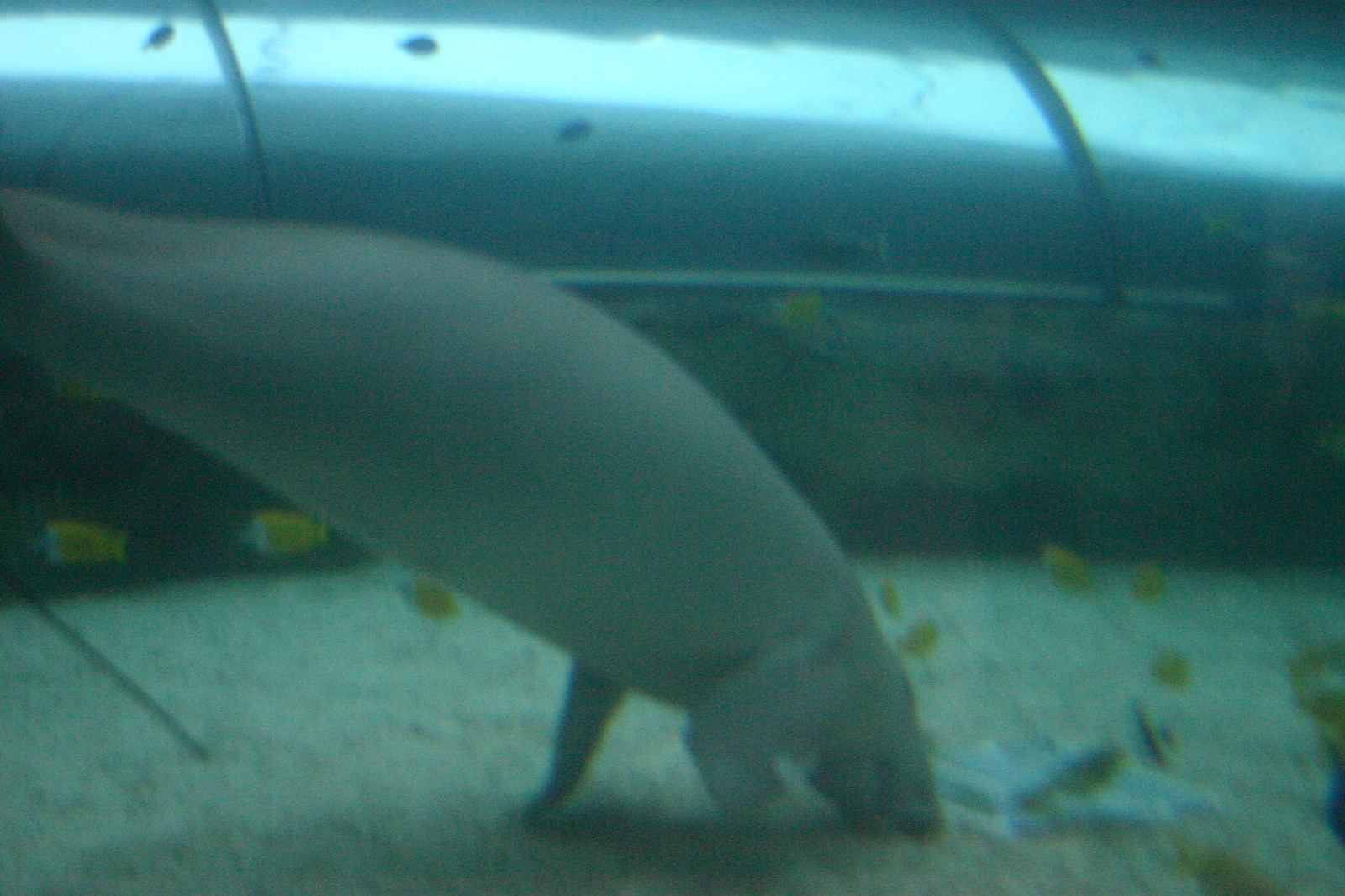The underwater scene depicts a large gray manatee positioned center frame, facing downward with its snout touching the sandy ocean floor as if it is eating something. The ocean floor is light brown, slightly blurred, creating a gentle contrast with the clear, algae-tinged water. In the background, spanning the entire width of the horizontally aligned rectangular image, a shiny gray cylindrical object resembling a submarine or large metallic pipe stretches from left to right. Surrounding the manatee are several small fish, including goldfish with white faces and others in shades of yellow and black, swimming in various directions, adding dynamic movement to the serene underwater setting.